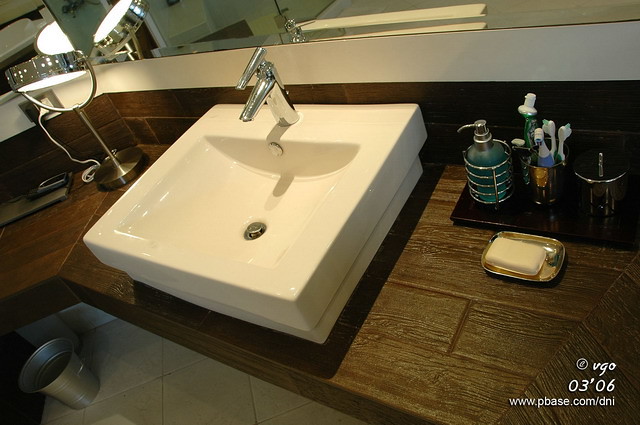The image depicts a meticulously designed bathroom counter area featuring a faux-wood finish in a rich brown color. The counter is uniquely tailored with angled segments: one stretching to the right and another extending to the left where a square sink with an arced basin is positioned. The sink is complemented by a sleek silver faucet equipped with a single handle. Above the counter, a backsplash matching the faux-wood pattern provides continuity, leading up to a white space that transitions seamlessly into a large, wraparound mirror.

On the counter, to the left of the sink, a small, plugged-in makeup mirror with built-in lighting commands attention. The right side of the sink is neatly arranged with a soap dish holding a bar of soap, a pump soap dispenser, a cup filled with toothbrushes, and an additional cup for miscellaneous items. In the bottom right-hand corner of the image, the text "www.pbase.com/dni03'06" is visible.